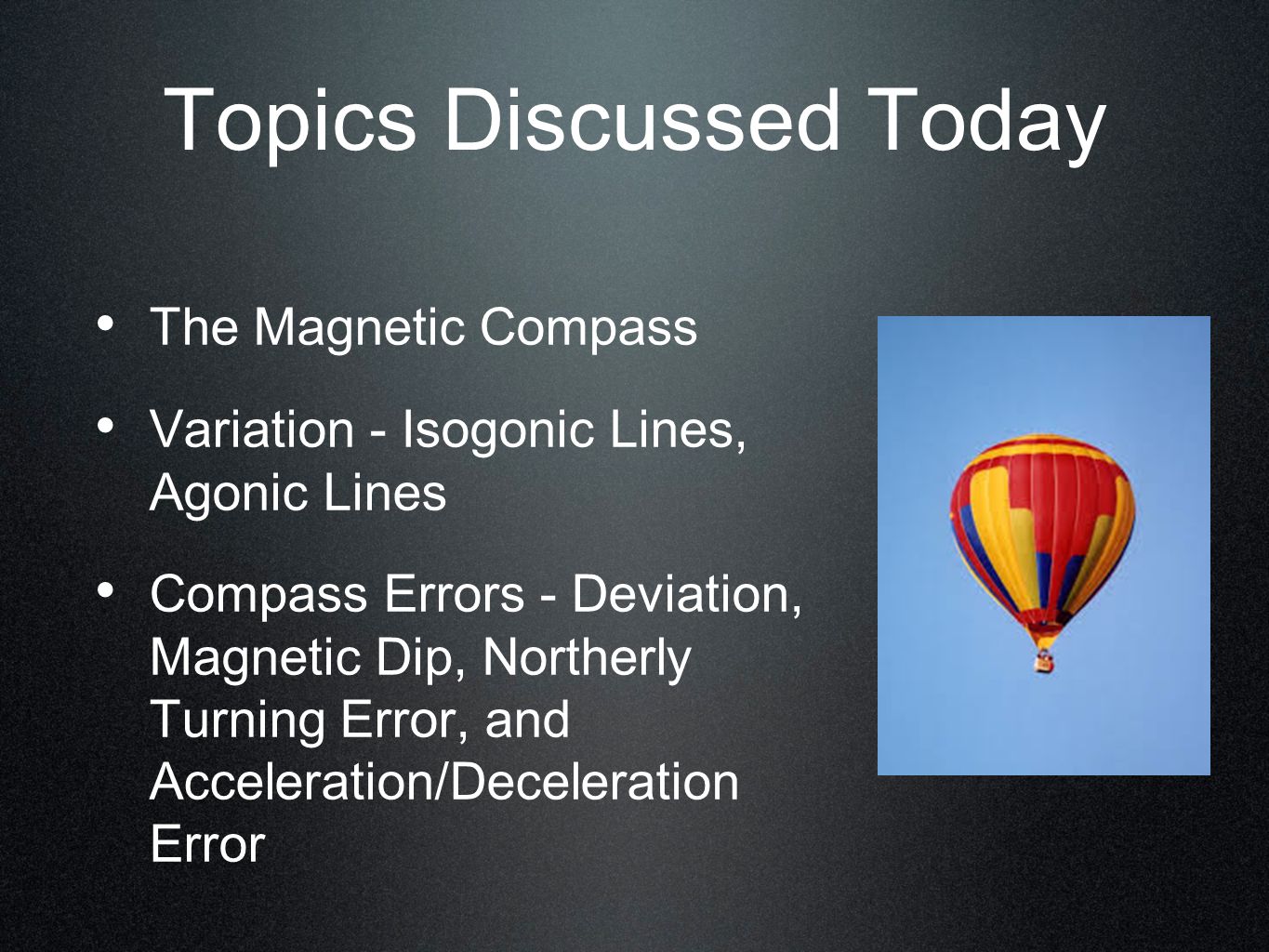The image depicts a slide from a PowerPoint presentation with a grainy black background. At the top, in large white text, it states "Topics Discussed Today." Below this title are three bullet points in smaller white text. The first bullet point reads "The Magnetic Compass," the second lists "Variation, Isogonic Lines, Agonic Lines," and the third enumerates "Compass Errors: Deviation, Magnetic Dip, Northerly Turning Error, Acceleration/Deceleration Error." On the right-hand side of the slide, there is a contrasting sky blue rectangle featuring a multicolored hot air balloon with vertical red, yellow, green, and blue stripes. Visible beneath the balloon is a basket, with an indistinct red element emerging from it. The image suggests a presentation on magnetic navigation and compass functionality, complemented by the colorful visual of the hot air balloon floating against a clear blue sky.